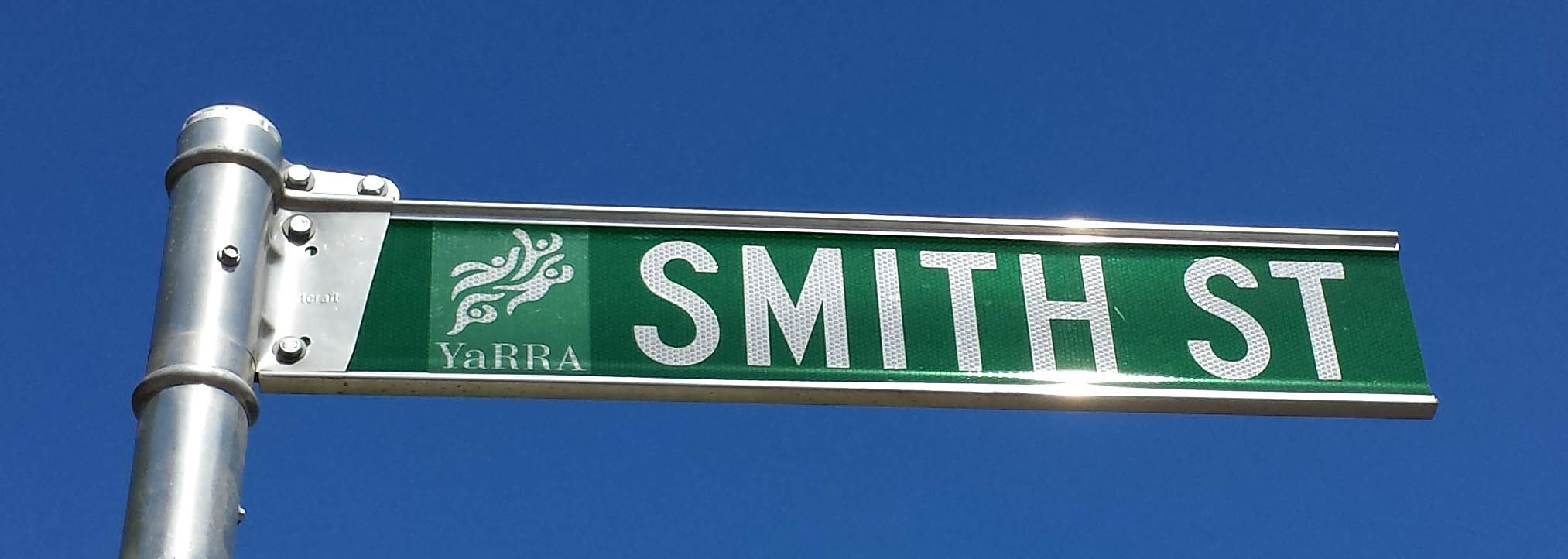This is a close-up, horizontal rectangular color photograph of a street sign against a dark blue, nearly unreal-looking uniform sky. The image focuses on the green street sign, showing only the very top of the shiny silver metal pole to which it is attached. The street sign itself is a narrow green rectangle, horizontally oriented, with white uppercase letters. It reads "Smith" followed by a space and "ST" in capital letters. To the left of "Smith ST," there is a smaller, lighter green vertical rectangle featuring the word "Yarra" in a mix of uppercase and lowercase letters, and above it, a logo depicting small, rounded, cartoonish figures that appear to be flying. The photograph captures the metallic sheen of the mounting bracket, highlighting the stark contrast between the vivid sign and the dark, almost surreal blue sky.